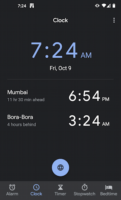This is a somewhat blurry color screenshot of a smartphone displaying a clock application, likely on an Android device. At the upper-center part of the image, the time "7:24 AM" is displayed in blue text, with "Friday, October 9th" directly beneath it in white. To the left of the main time display, "7:24" appears again in white in the top-left corner, accompanied by a small, squarish white icon. Above the central time display, the word "Clock" is written in white text.

In the upper-right corner, typical status icons are visible: a Wi-Fi signal, cellular signal strength, and a partially discernible battery indicator, along with another indiscernible icon. The screen has a black background, making these white elements stand out sharply.

Moving downward, there are three buttons positioned to the right of the "Clock" label. Below these buttons, two world clock entries are listed: "Mumbai, 6:54 PM" and "Bora Bora, 3:24 AM," with some additional text beneath each that is not legible due to the blurriness. A very thin horizontal line separates these elements from the rest of the screen.

Near the bottom center of the image, a round blue button can be seen, though its purpose isn't clear from the context. The very bottom part of the screenshot contains a slightly greyer band featuring a series of icons which likely represent the following functions (from left to right): alarm clock, main clock, timer, stopwatch, and a person with a bed icon (which could relate to a sleep or bedtime feature).

Overall, the screenshot depicts the interface of a mobile clock app with various world clocks and standard clock functions readily accessible via icons at the bottom of the screen.